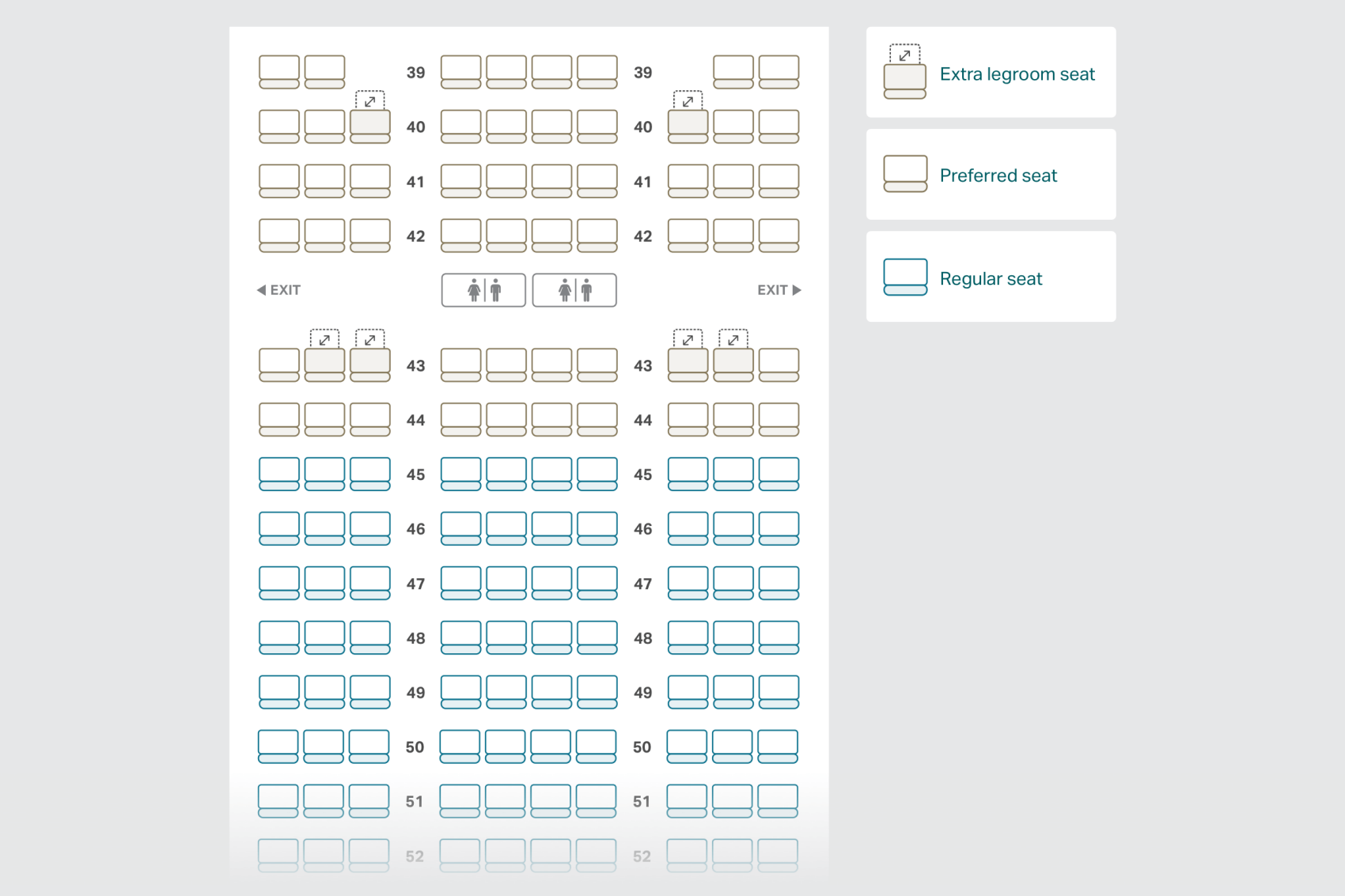In this image, the design features a light background encompassing the entire layout. On the left side, there are multiple squares arranged in a grid format. The grid starts with rows of three squares on the left, then transitions to rows of four squares in the center, and concludes with rows of three squares on the right. Each square in the top rows is outlined in gray, while the squares in the bottom rows are outlined in blue. These squares are labeled with numbers sequentially: 39, 40, 41, and 42 on the first row; 43, 44, 45 (where the blue outlines begin), 46, 47, 48, 49, 50, and finally 51, with 52 being faded at the bottom.

To the right of the grid, there are three white rectangles stacked vertically, each labeled to indicate different seating options. The top rectangle is labeled "Extra Legroom Seat," the middle rectangle is marked "Preferred Seat," and the bottom rectangle is titled "Regular Seat." Additionally, on the left and right sides of the grid, there are options labeled "Exit." In the center of the image, towards the bottom, there are icons depicting two people.

Overall, the image is a detailed layout diagram, depicting seating options and exit points, likely for an auditorium, theater, or transportation seating plan.